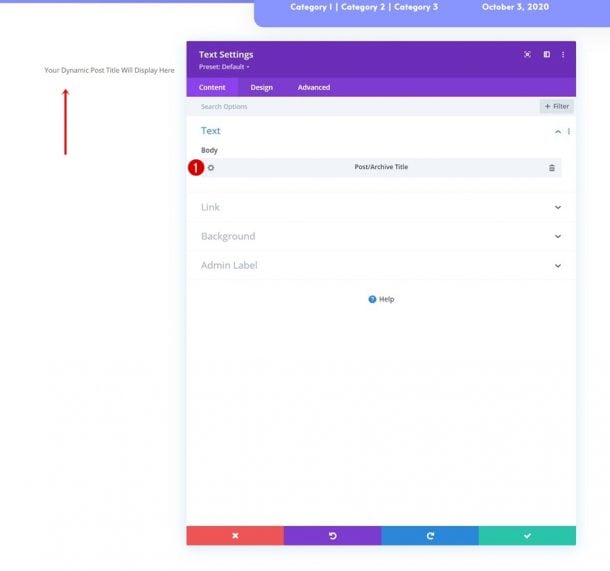The screen displays an intricate interface layout with numerous sections. At the very top, a thin blue line runs horizontally across half the screen, transitioning at the midpoint into a wide blue ribbon. Inside this ribbon, bold white text labels three categories: "Category 1," "Category 2," and "Category 3," followed by "October 3rd, 2020" on the right side. Below this wide blue ribbon is a vertical rectangular box highlighted by a bright purple ribbon at its top. The purple ribbon displays "Text Setting" in white text, with the words "Preset Default" in italics just beneath it.

Further down, there is a lighter purple banner bearing the terms "Content," "Design," and "Advanced" in white text, arranged from left to right. Underneath this banner, a very light green banner reads "Search Options" in gray text. 

Continuing below on a white background, the word "Text" appears in bright blue, with the word "Body" underneath it in gray text. A light blue banner runs horizontally across the page, the center of which contains the text "Post / Archive Title" in gray. To the left of this banner, a small red circle with the number "1" inside is prominently displayed. Following this section on a white background, three terms are listed sequentially in light gray text: "Link," "Background," and "Admin Label."